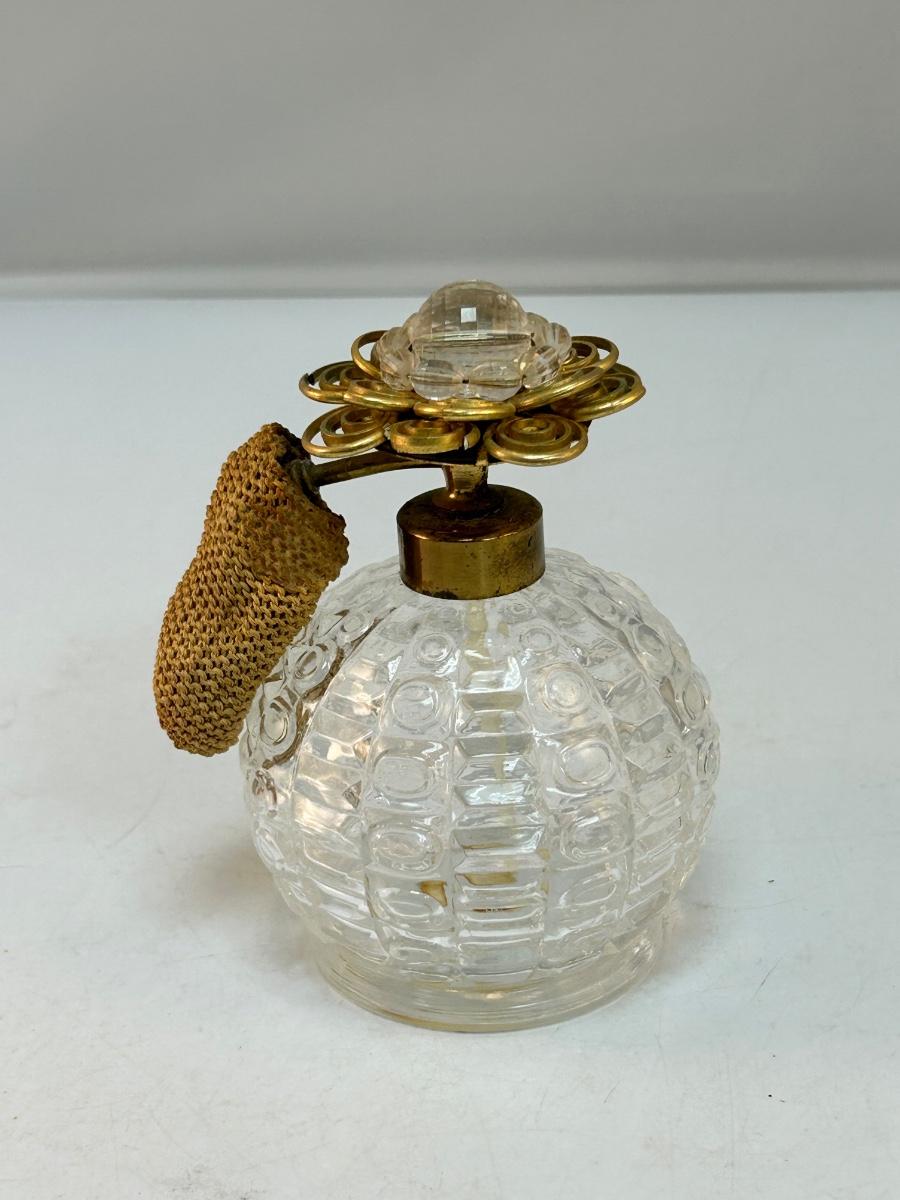This image showcases an antique crystal perfume bottle, characterized by its intricate and elaborate design. The base of the bottle is completely round, with a pattern of vertically aligned circles and ovals, giving it a sophisticated, globe-like appearance. The crystal structure is complemented by a darker, brass-like gold lid that appears slightly tarnished, adding to its vintage charm. At the top of the lid is a very ornate, floral-shaped handle with multiple layers, also crafted from the same brass-like material. On top of this handle, there's a clear glass decoration, akin to the material of the bottle itself. Hanging off the far left side of the cap is a knitted cover, resembling a small brown bag or sock, obscuring where the perfume might be dispensed. The entire ensemble rests on a white surface, against a white backdrop, enhancing the elegant and historic aesthetic of this piece.